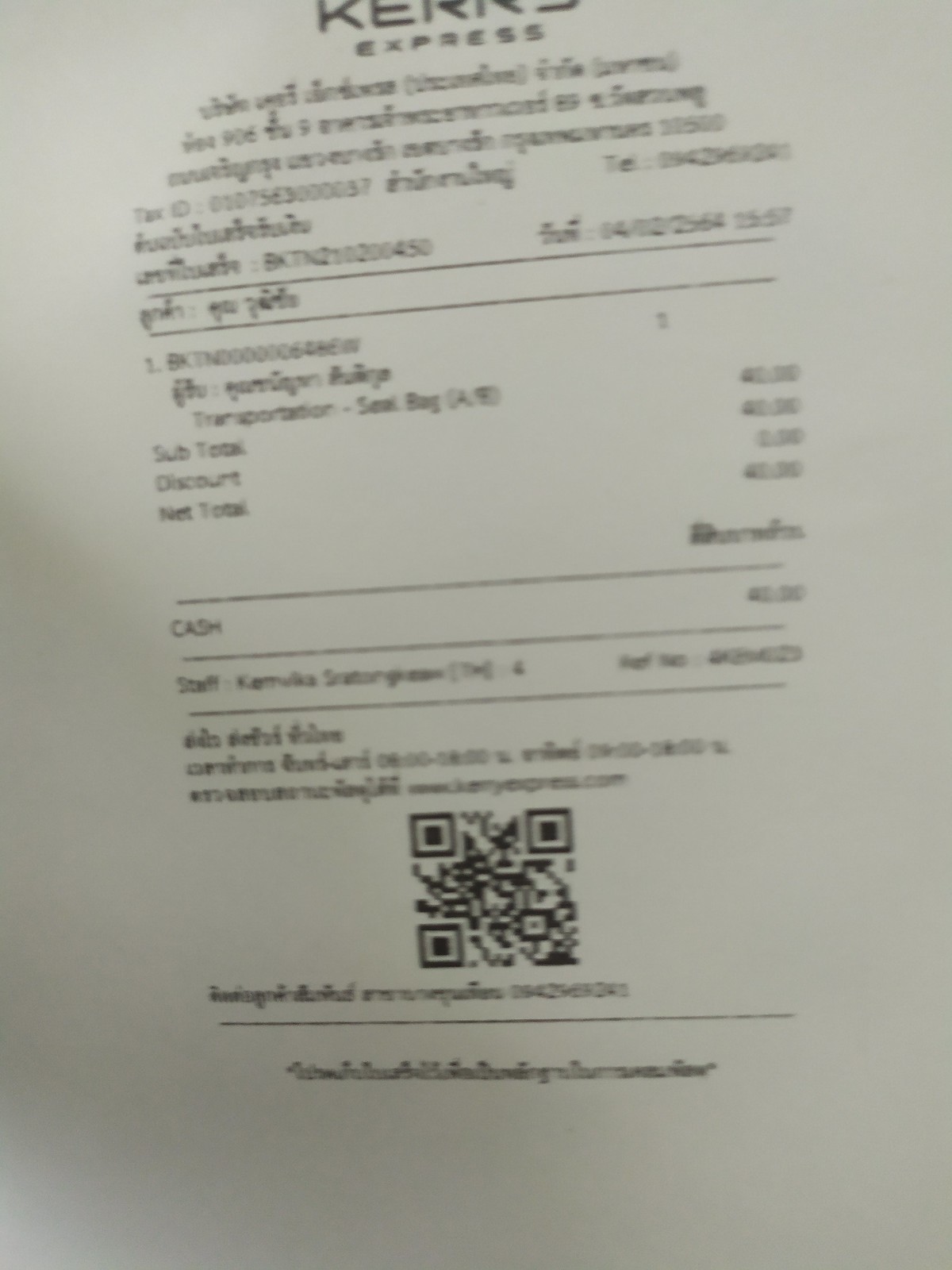The photograph depicts a somewhat blurry receipt issued by an establishment named "Kurz Express." Despite the unclear image quality, certain details are discernible. The receipt appears to be dated, albeit ambiguously, as either 1402 or perhaps 2064; such dates seem impossible, suggesting a typographical error. The itemized purchases are indiscernible, but the total amount is legible, showing a cash payment of $41.30. The receipt features black text printed on a white background and includes the name of the staff member who processed the transaction, as well as a QR code located at the bottom.